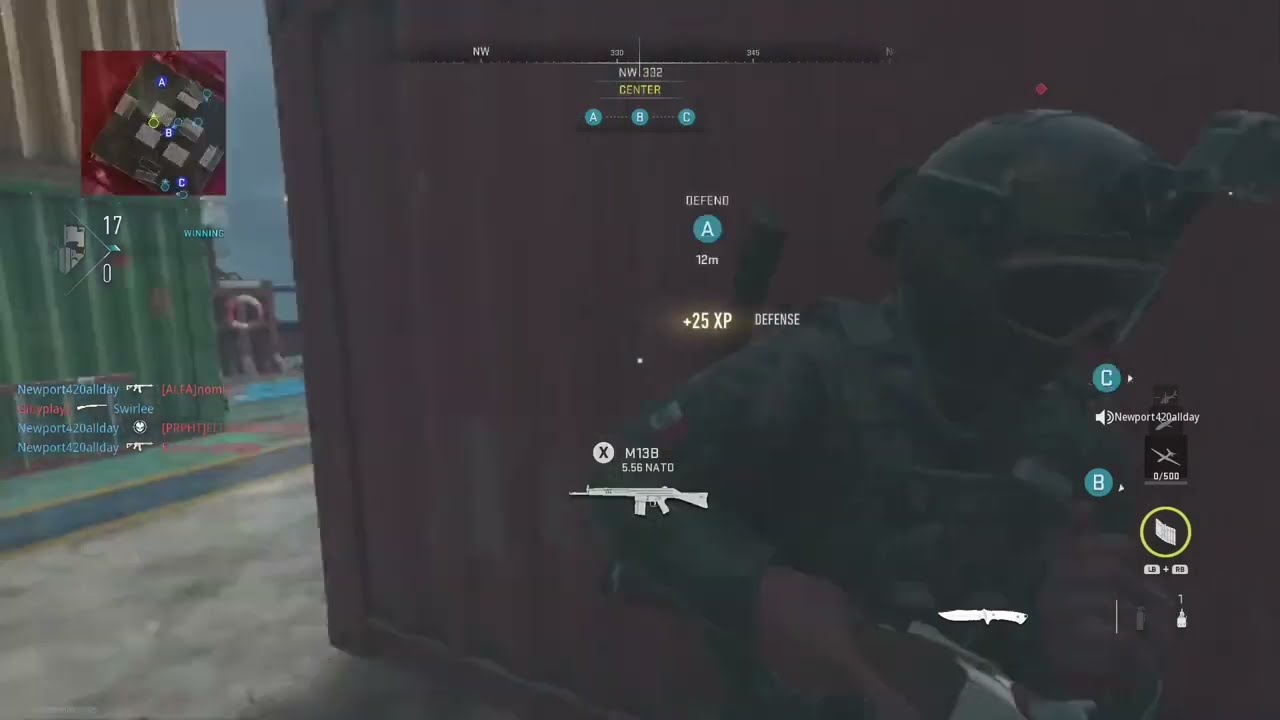This image is a detailed screen capture from a first-person shooter video game. On the right side of the frame, we see another player character, prominently featured from the waist up, dressed in green camouflage gear, including a military-style helmet, armored vest, and black goggles. The character is holding a weapon, presumably a gun, and seems to be in motion towards the right side of the screen.

In the background, there is a large rust-colored shipping crate dominating the right-hand side of the scene. To the left, further back, are additional crates, including a yellow one stacked on top of a green one. The ground appears to be gray pavement, and in the distance, a gray-blue sky can be seen.

Overlaying the game scene are several interface elements: a mini-map in the upper left corner, a compass at the top center displaying a northwest direction, and weapon select icons in the bottom right which include a picture of a knife. Additionally, player usernames are displayed on the left side, and various control icons, like letters C and B in circles and the letter X naming a gun, are also visible. The intricate layout and interactive elements underscore the immersive gameplay environment.